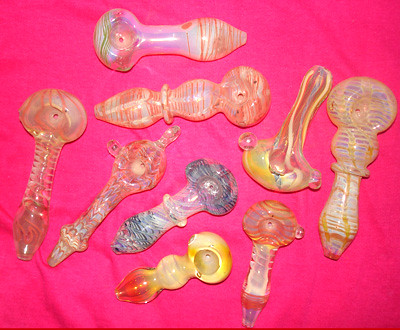This image captures a collection of nine distinctive glass pipes, possibly used for smoking marijuana, artistically arranged on a vibrant pink sheet. Each pipe is unique in shape and size, with some featuring spoon-like curves and dips, while others are more elongated with wider circular bases. The glass pieces are not just functional but also highly decorative, showcasing vivid colors such as yellow, teal, and orange, with intricate patterns and streaks. The overall composition suggests an artistic display, possibly for sale or collection, highlighting the craftsmanship and creativity often associated with glass blowing.